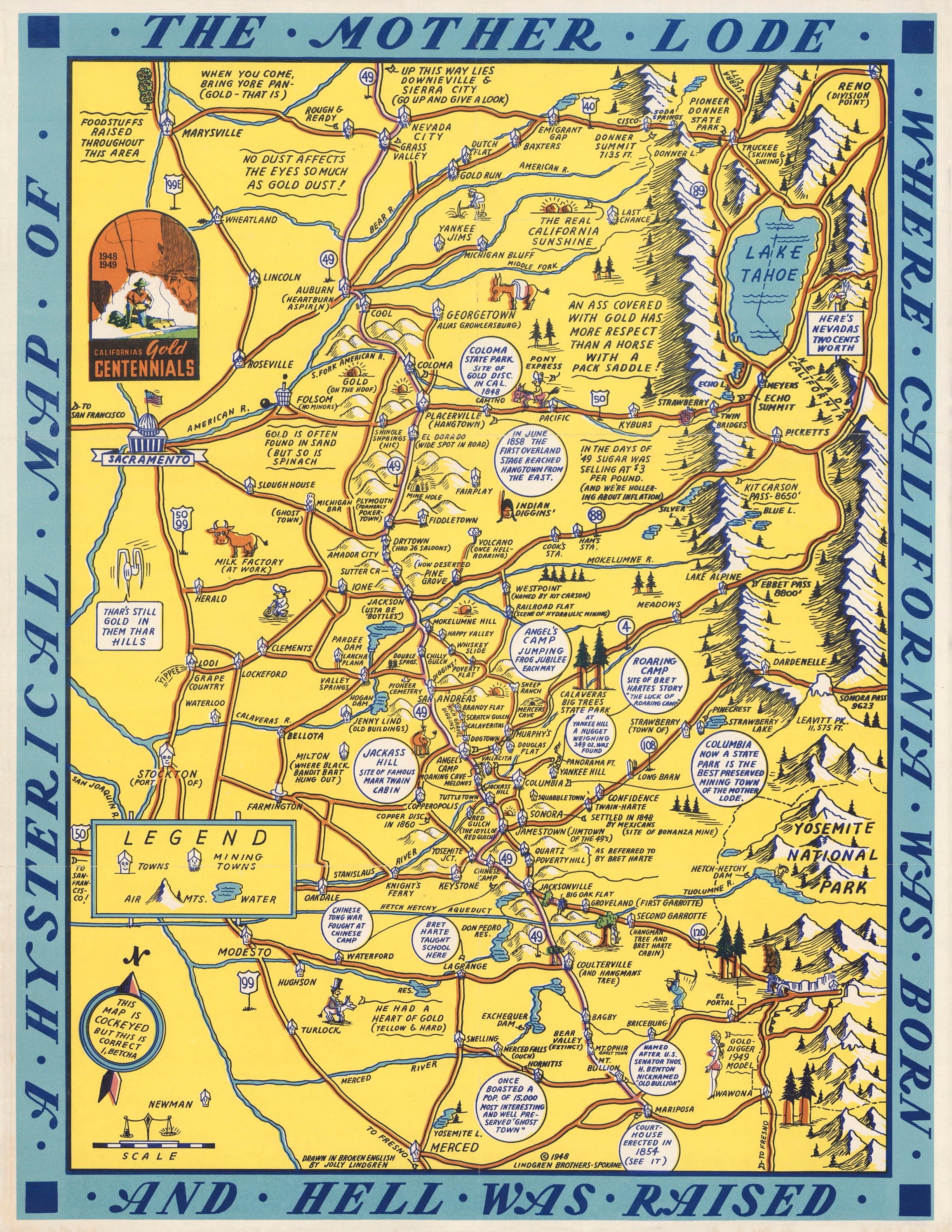This image depicts an old-style illustrated map of California, titled "The Mother Lode," which is surrounded by writing on all four sides stating: "A Hysterical Map of the Mother Lode Where California Was Born and Hell Was Raised," with a period between each word. The map, framed by a light blue border with navy blue squares at each corner, features a yellow background and various annotations in black. Key landmarks such as Sacramento, Lake Tahoe, and Yosemite National Park are included, along with numerous highways, interstates, and mining towns. The legend in the bottom left details towns, mining towns, mountains, and bodies of water, emphasizing the significance of gold mining. The map also includes a logo in the top left corner reading "California's Gold Centennials" and is dated 1948, reflecting both the historical and cultural aspects of California's gold mining era.